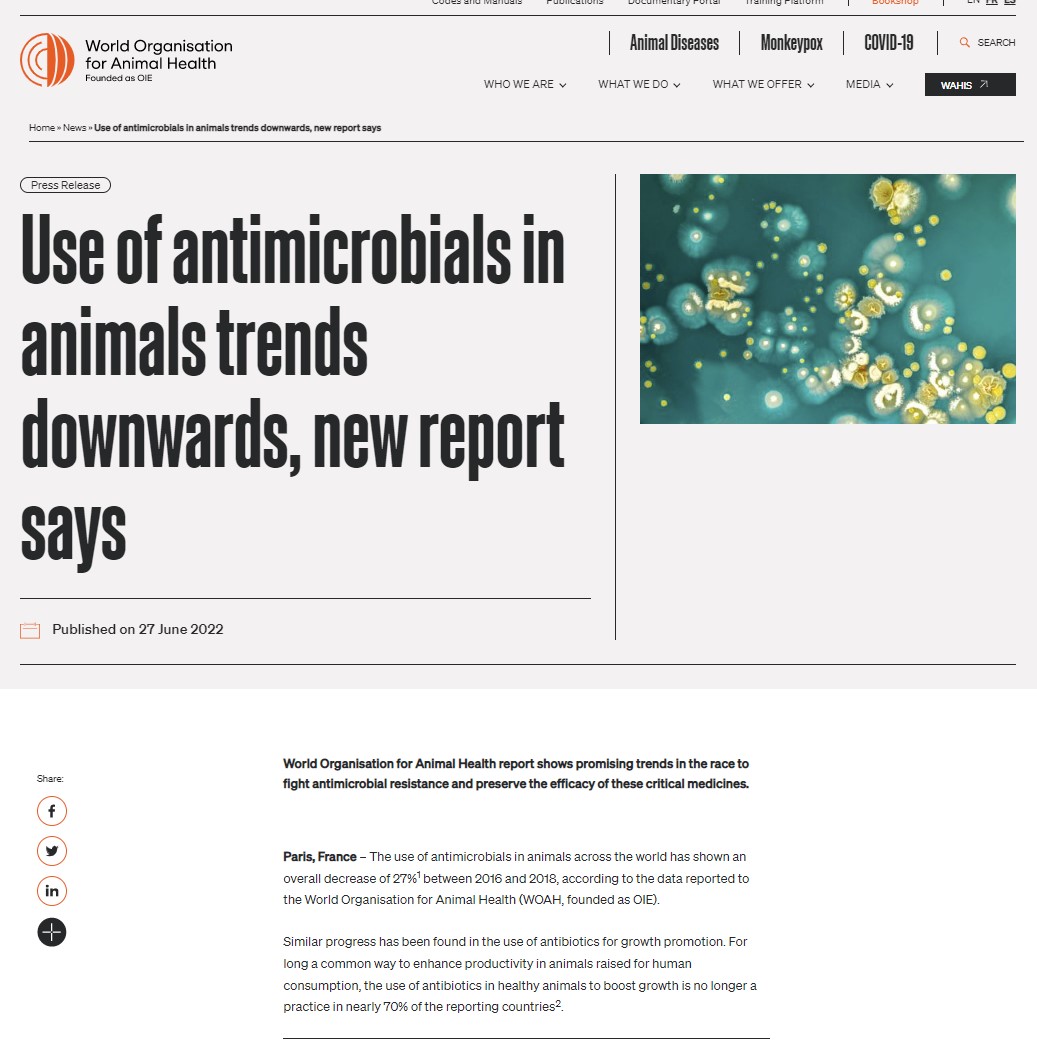Here is a descriptive and cleaned-up caption for the image:

---

Screenshot of a newspaper article published on June 27, 2022, titled "Use of Antimicrobials in Animals Trends Downwards, New Report Shows." The article, published in Paris, France, by the World Organization for Animal Health, discusses encouraging trends regarding the reduced use of antimicrobials in livestock. The report highlights the organization's efforts in combating animal diseases such as monkeypox and COVID-19. A vertical social media sharing toolbar is visible, featuring buttons for Facebook, Twitter, LinkedIn, and an additional sharing option. The article is accompanied by an illustrative image of bacteria.

---